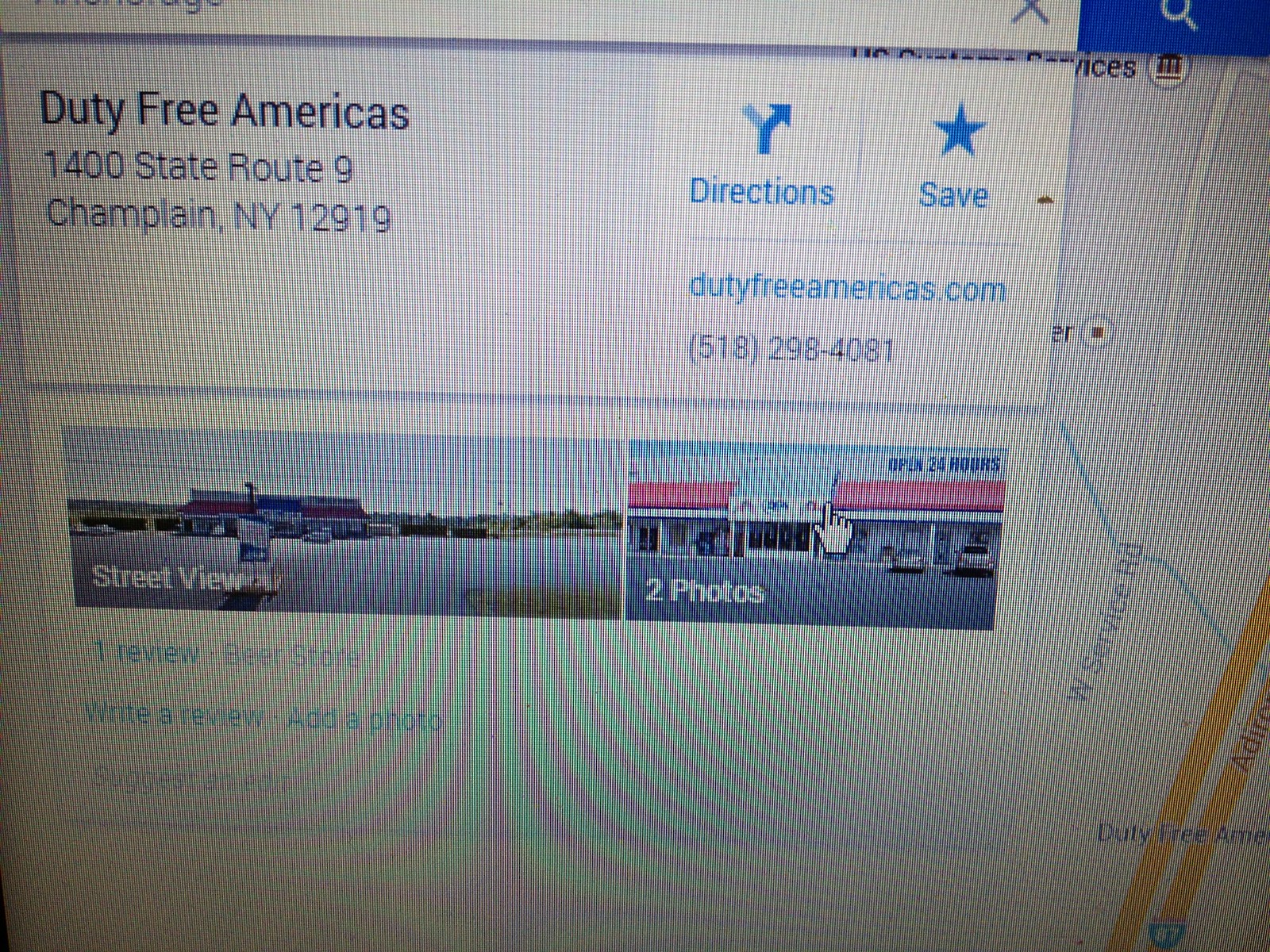This photograph captures a computer screen displaying a Google Maps page with directions to Duty Free Americas, located at 1400 State Route 9, Champlain, New York, 12919. The screen shows the distinctive horizontal lines typical when photographing a display. In the upper left corner, the name "Duty Free Americas" is prominent, accompanied by the address, and options for directions and saving the location. The website dutyfreeamericas.com and phone number (518) 298-4081 are provided. A box on the screen displays additional information including a street view image of the store, two photos, and options to write a review or add a photo. Adjacent to this informational box, there's a small map showing part of a service road and nearby highways, slightly visible behind the overlay. The top right corner of the box includes an 'X' option to close it, potentially revealing a full view of the map behind it.